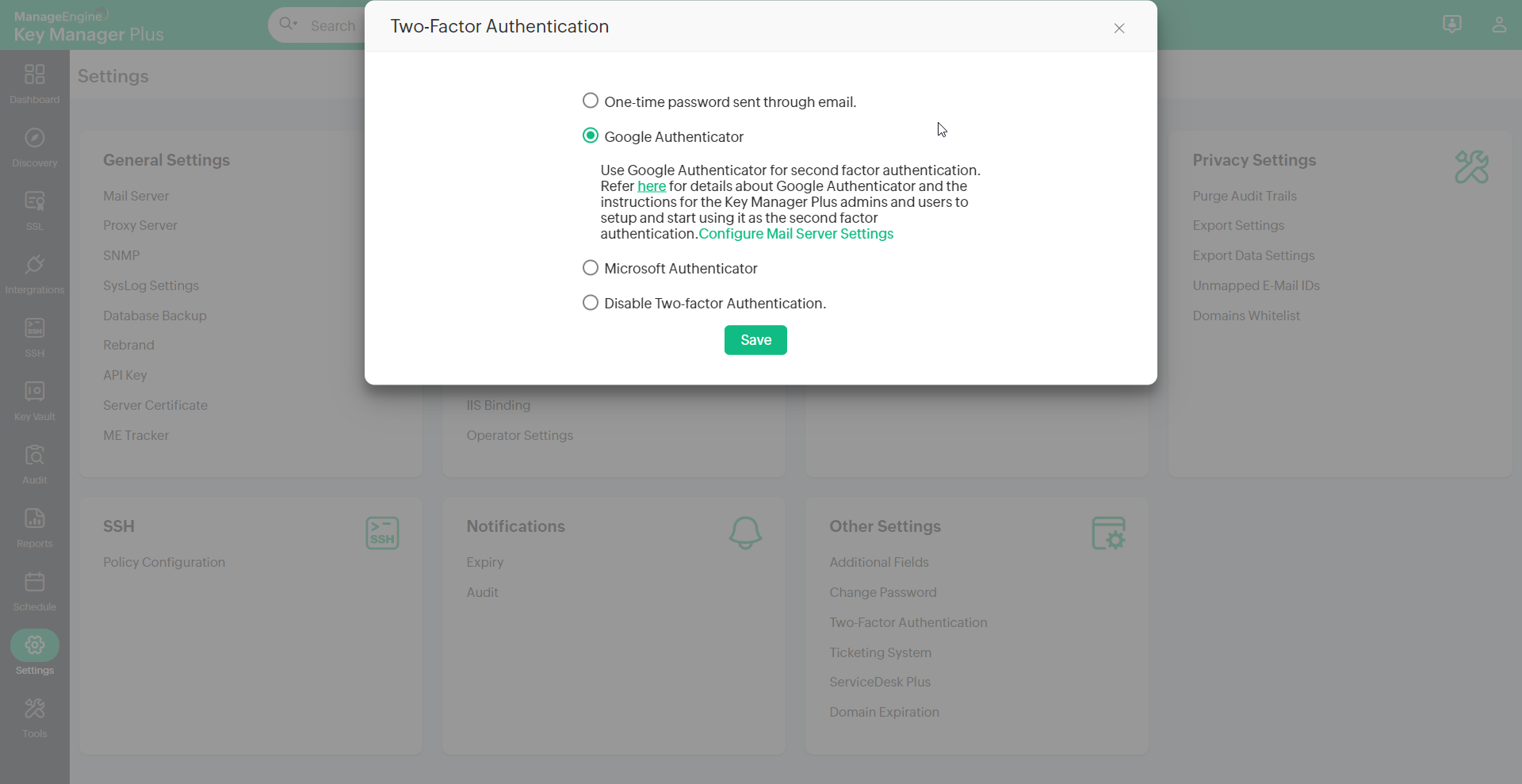**Descriptive Caption:**

The ManageEngine Key Manager Plus interface is presented on a well-organized UI layout. The screen is divided into three distinct panes. On the far left, a vertical toolbar with a black background and white text displays key navigation options such as Dashboard, Discovery, Audit, Reports, Schedule, and Settings. The middle, slightly narrower pane focuses on the application's settings. In this particular view, the user has navigated to the Settings section, revealing further options including Two-Factor Authentication, User Management, General Settings, and Privacy Settings. Within the Two-Factor Authentication settings, the user can choose from four options for securing their account: one-time password via email, Google Authenticator, Microsoft Authenticator, or disabling two-factor authentication. The selected option, Google Authenticator, is highlighted and will be used for second-factor authentication. There are prompts to configure mail server settings to facilitate the setup and ensure secure access.